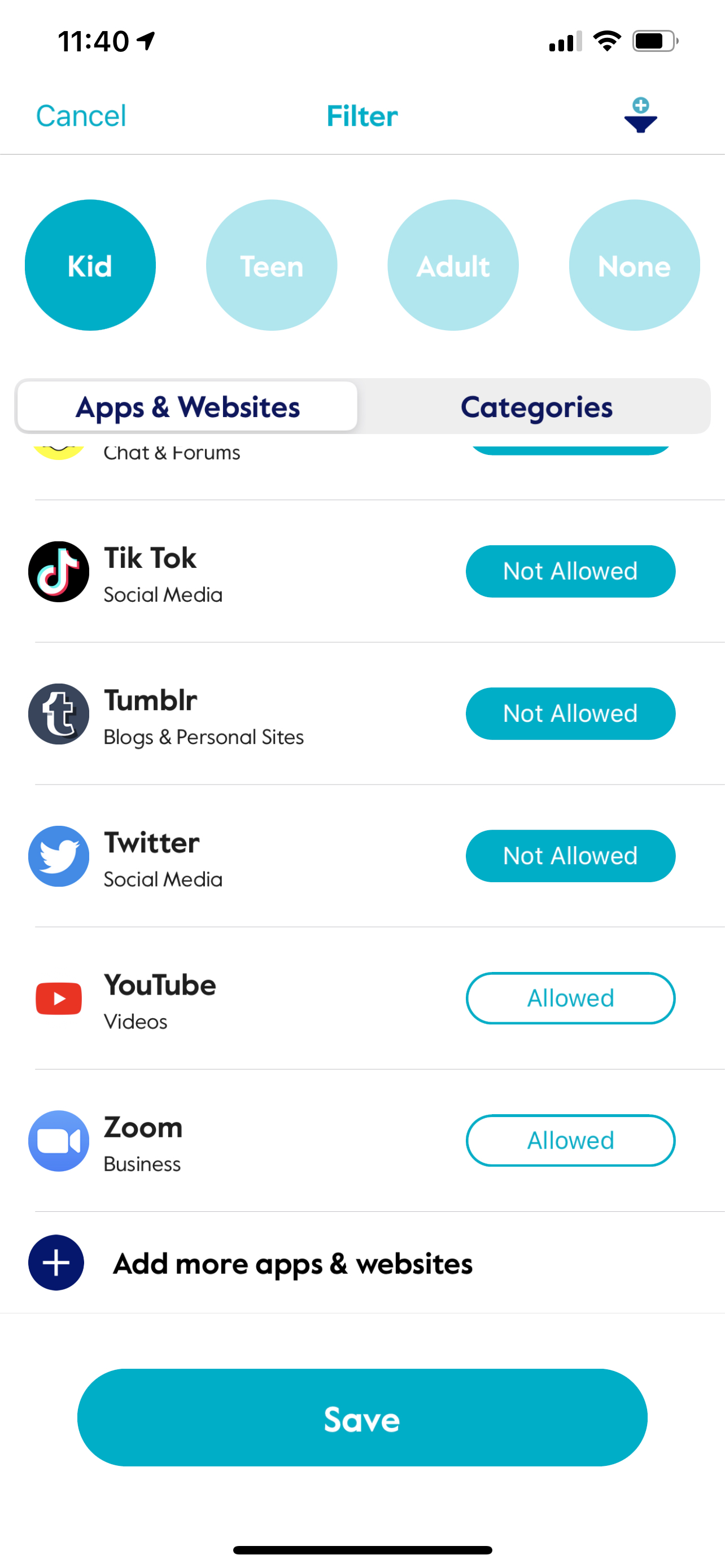The image depicts a smartphone displaying a website interface with a filter feature. The status bar at the top of the screen shows the time as 11:40, a nearly full battery, and a stable internet connection. 

At the center, "Filter" is prominently written in blue, flanked by a blue "Cancel" button on the left. Below the filter title, there is an icon resembling an upside-down triangle with a small circle on top. Just beneath this icon are large, turquoise blue circles labeled "Kid," "Teen," "Adult," and "None," with the "Kid" option highlighted in a darker blue.

Continuing down the screen, there's a section titled "Apps and Websites Categories." Under this heading, the first category is partially visible, with the name cut off. Subsequent categories listed include "TikTok" marked as "Not Allowed" under "Social Media," "Tumblr" labeled as "Blogs and Personal Sites," also "Not Allowed," "YouTube" marked as "Allowed" under "Videos," and "Zoom" marked as "Allowed" under "Business." The "Not Allowed" categories are indicated with teal circles, whereas the "Allowed" categories are shown with white circles trimmed in teal.

Towards the bottom, there's a plus sign enclosed in a navy circle, next to the text "More Apps and Websites." Concluding the interface is a teal "Save" button with white lettering, followed by a black bar at the very bottom of the screen.